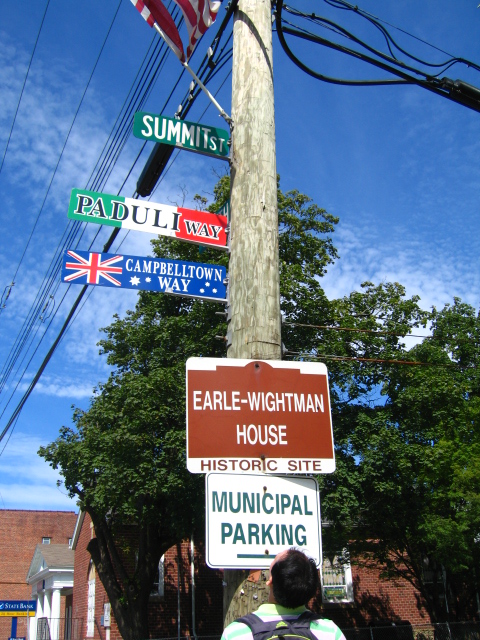In the foreground of this color photograph, a man with black hair wearing a white short-sleeved polo shirt with green stripes and a backpack stands at the base of a telephone pole, facing away from the camera and looking up. The central telephone pole features multiple signs and wires. Starting from the bottom, the first sign reads "Municipal Parking" in green font on a white background, with an arrow pointing to the right. Directly above it is a brown sign labeled "Earle Whiteman House Historic Site." Higher up the pole is a green street sign for "Summit Street." Additional street signs are mounted around the pole: "Paduli Way" in the colors of the Italian flag (green, white, and red), and "Campbelltown Way," which is blue with a Union Jack and several white stars. The top of the pole is adorned with an American flag fluttering in the breeze. In the background, a mix of trees and a brown brick building—a State Bank, partially visible—can be seen under a blue sky with scattered clouds. The image captures a web of utility wires extending from the pole, adding a sense of urban complexity to the scene.